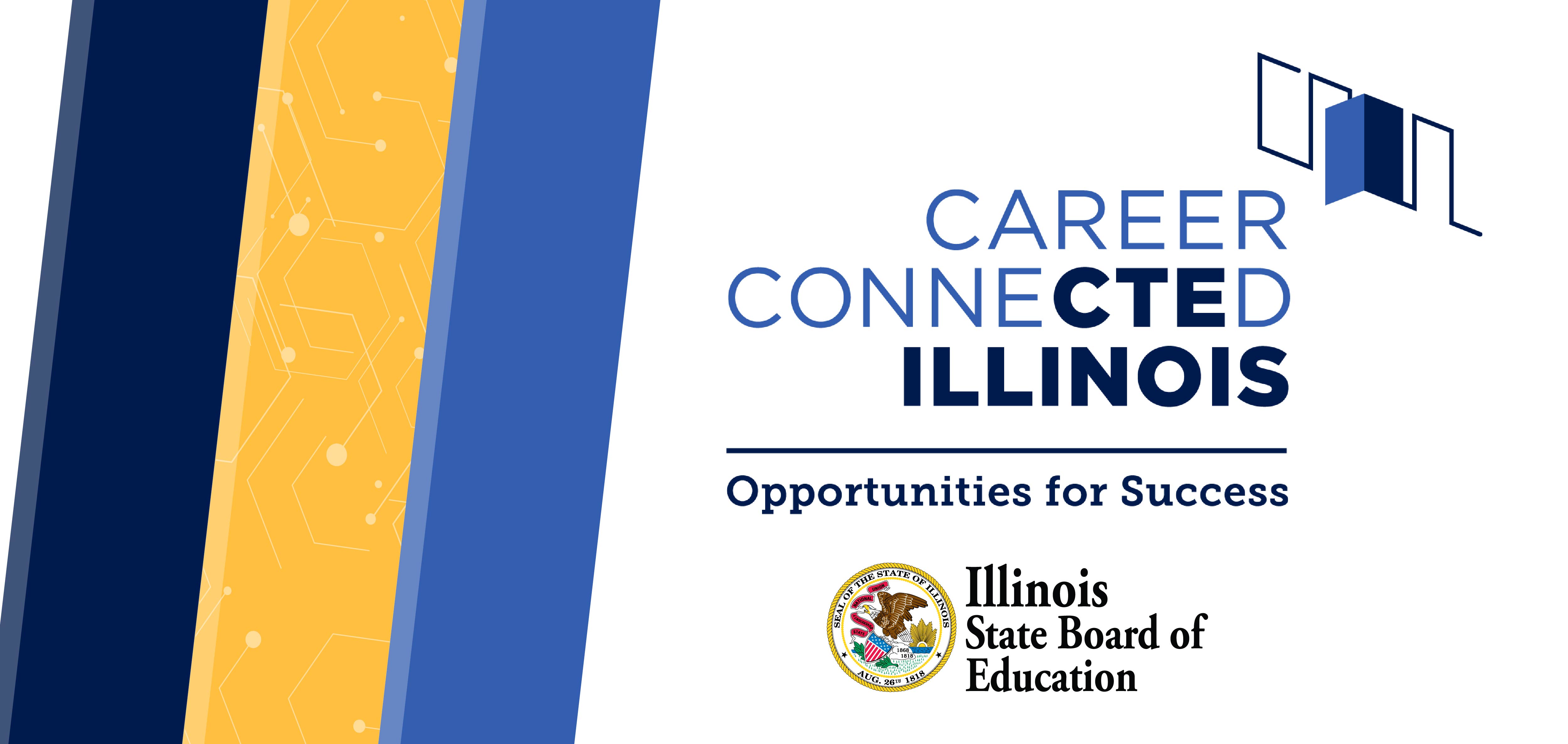The image depicts a promotional banner with detailed design elements and informative content. On the right side of the banner, a white section houses all the essential information.

In the top right corner, there is a distinctive logo composed of angular blue lines resembling door frames. One segment of the logo features a door, illustrated with a blue shape and a dark blue interior, creating a striking visual effect.

Below the logo, three rows of heading text are displayed prominently. They read "Career Connected Illinois," with specific emphasis on parts of the words. "Career" and sections of "Connected" are highlighted in a vibrant blue color, while "CTE" in "Connected" and "Illinois" are in a bold, dark blue.

A dark blue line separates the heading text from the subheading, which states "Opportunities for Success" in a serif font. Beneath this subheading is a badge icon, presumed to represent the state of Illinois. The badge features a bird, likely a bald eagle clutching a snake above some plants, reminiscent of the imagery found on the Mexican flag, but distinctly different. The badge is bordered in gold.

To the right of the badge, the text reads "Illinois State Board of Education" in a serif typeface, with the color appearing to be either dark blue or black.

The left portion of the banner features decorative diagonal sections that add an aesthetic flair. The first section is a royal blue with a sliver of a lighter blue border. The middle section is yellow, adorned with a lighter yellow, almost white, scientific or technical pattern. The leftmost section is dark blue, complemented by a lighter shade of the same dark blue.

Overall, the banner is wide and not very tall, combining detailed graphics and well-structured information.